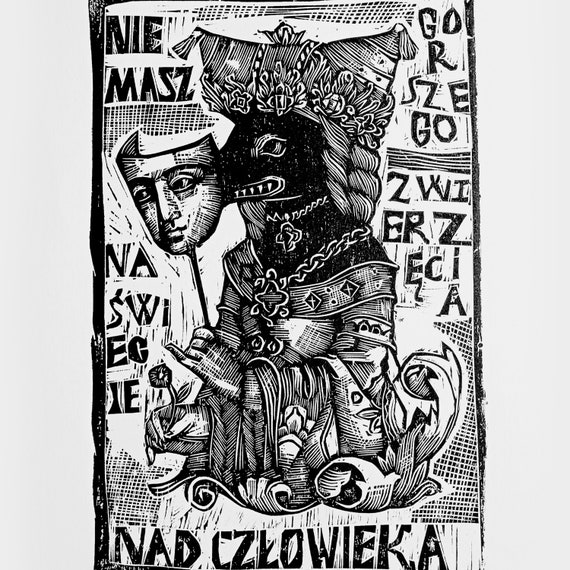The image is a striking black-and-white vertical poster with a light gray background. At the center of the poster, there is a detailed illustration of a dog, which appears to be anthropomorphic, seated in a human-like posture. The dog is extravagantly dressed, featuring a large chain around its neck and a massive medieval-style headdress with braids coming out from beneath it. This headdress gives an imposing and regal appearance. The creature's hands are human-like and it holds a black rod with a theatrical mask of a male human face, reminiscent of the BAFTA award mask. There is intricate detail in the robes and outfit, which includes heavy chains and elaborate gold-like patterns, adding to the grandeur and surreal quality of the image. Surrounding the illustration, there is text in a non-English language: the bottom prominently displays "NAD CZLOWIEKA", while the upper left corner reads "NIE MASZ", and the upper right section features a staggered arrangement of the words "GRO GORSZEGO ZWI ERZ ECI A". The artwork gives off a surreal, almost grotesque blend of human and animal elements, capturing a compelling visual that is both eerie and fascinating.